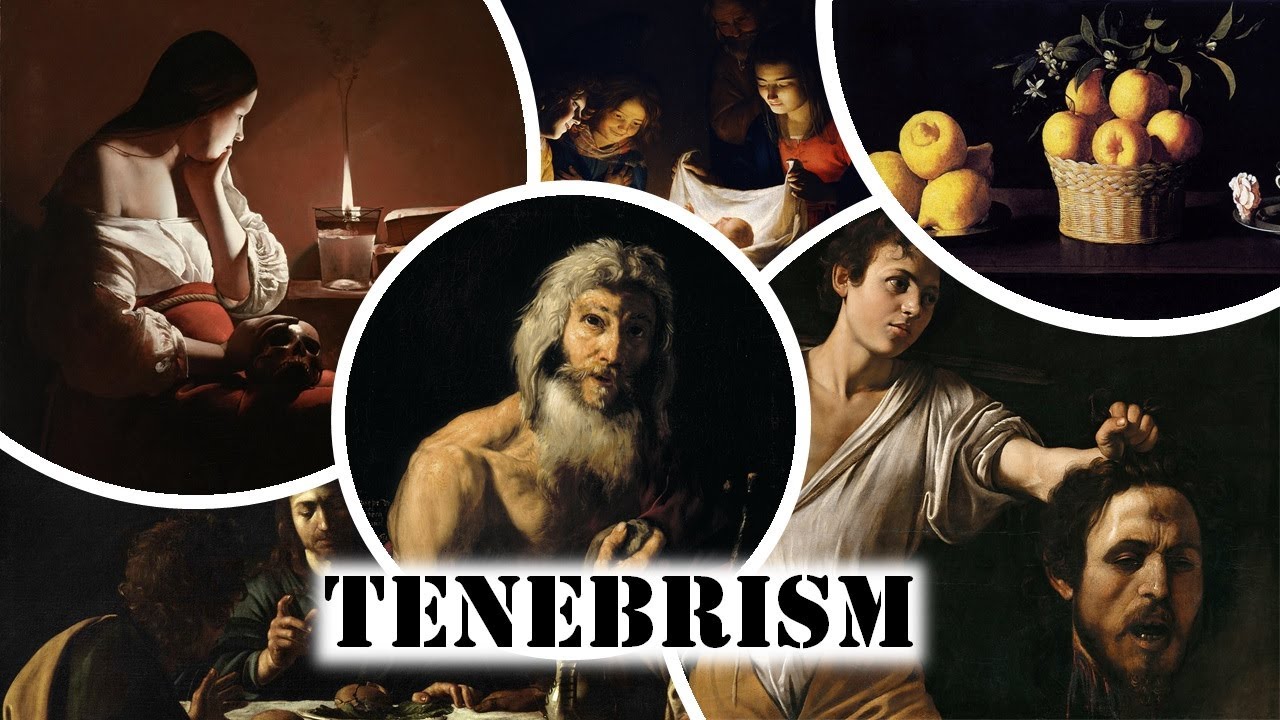The dark, enigmatic image is composed of four distinct sections, each framed by white outline circles against a shadowy background. Across the bottom center, a white banner prominently displays "Tenebrism" in black capital letters. 

In the top left circle, a young woman with dark hair sits in a chair, her face partially illuminated by the flickering flame of a candle she is intently gazing at. She wears an off-the-shoulder Spanish-style top paired with a visible red skirt, set against a brown backdrop.

The center circle features an older man with shoulder-length graying hair, a graying mustache, and a short beard. His tan or beige outfit contrasts with his somber expression and the detailed texture of his hair.

To the top right, a wicker basket filled with yellow apples or pears is depicted on a dark background. Beside the basket, a couple of lemons are stacked, adding a touch of brightness to the composition.

Finally, the bottom right circle reveals a dramatic and unsettling scene: a man with an open white shirt extends his left arm. Grasped by the hair, he holds a severed head, its eyes partially closed, and adorned with a dark mustache and beard, dangling ominously in the shadowy space.

This intricate and striking composition masterfully employs chiaroscuro to evoke intense emotional and visual impact.